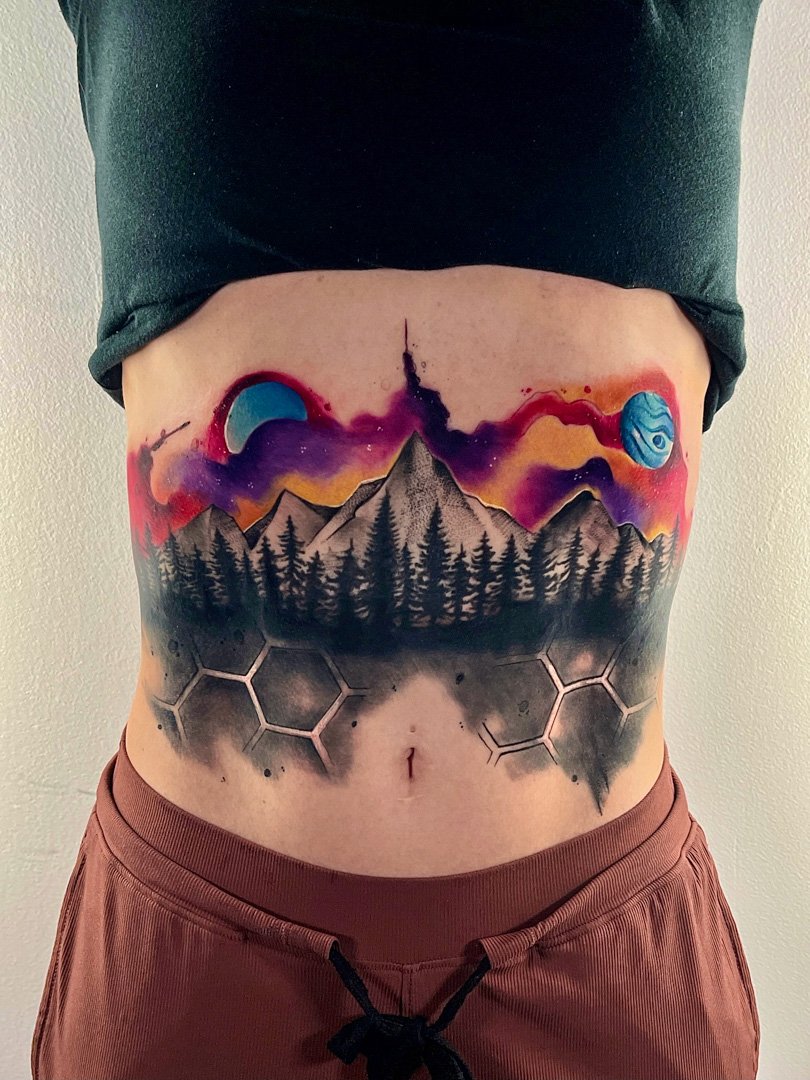This image features a woman's midsection showcasing an elaborate tattoo. She is dressed in a black tank top rolled up to reveal the artwork, and brown sweater lounge pants with a black drawstring tied at the waist. The background is white.

The tattoo spans her stomach from below the chest to above the belly button, which is marked by a thin vertical line. The intricate design begins at the top with vibrant swirls of orange, red, purple, and yellow hues. On the left, there's a grayish-blue crescent moon, while to the right, a blue planet with wavy lines is depicted.

Below these celestial elements, a mountain range emerges, featuring a prominent central peak surrounded by smaller mountains. Dark, black pine trees are etched in front of the mountains, and the design transitions into honeycomb shapes at the bottom, highlighted with white outlines and dark gray shading.

This comprehensive tattoo blends vivid colors and complex shapes, creating a stunning, multi-layered scene on the woman's stomach.